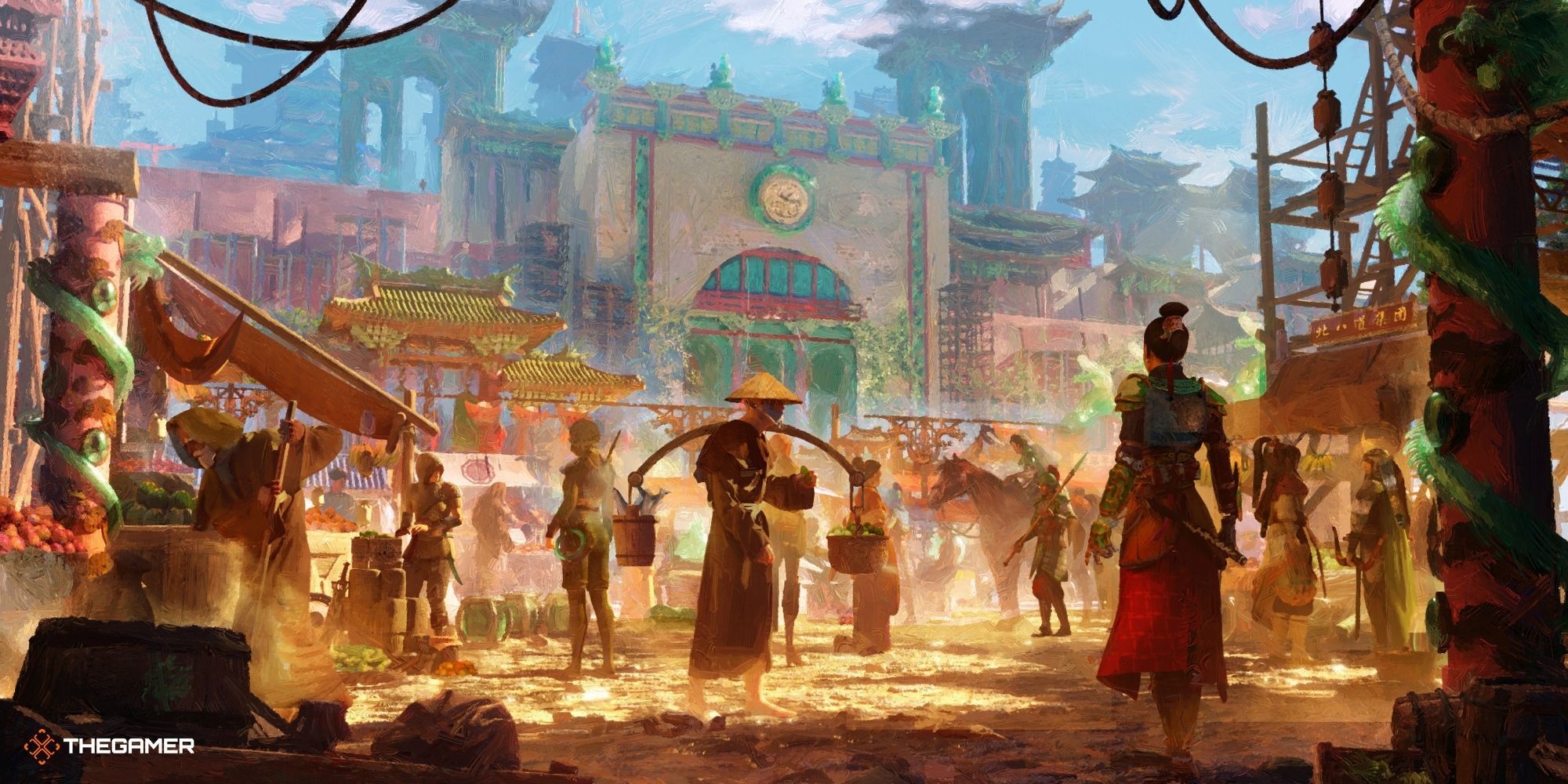The image depicts a vibrant concept art scene from a video game, set in an ancient, oriental-style marketplace. The marketplace, brimming with activity and various characters, features a blend of traditional and modern architectural elements, including towering skyscrapers and temple-like structures. Prominently featured on the right side, facing away from the viewer, is the likely main character—a female warrior clad in intricate armor with brownish metal arms and a shoulder pad on the left. She sports a red skirt and has her hair bun tied neatly at the back. 

In the bustling courtyard, an old man wearing a long brown robe and a conical straw hat strides across the scene, carrying buckets on either end of an arced piece of wood slung over his shoulder. Nearby, a woman with a bow stands at the far right, and a guard with a spear keeps watch. An array of market stalls populates the scene, offering various goods, with some attendants donning traditional rice hats. To the left, among pagoda-style roofs, a noteworthy column with green eyeballs and a snake wrapped around it can be spotted.

In the bottom left corner of the image, a red diamond shape with an 'X' or cross inside catches the eye, adjacent to the title "The Gamer" written in all-capital, white text, reinforcing the image's connection to the video game world.